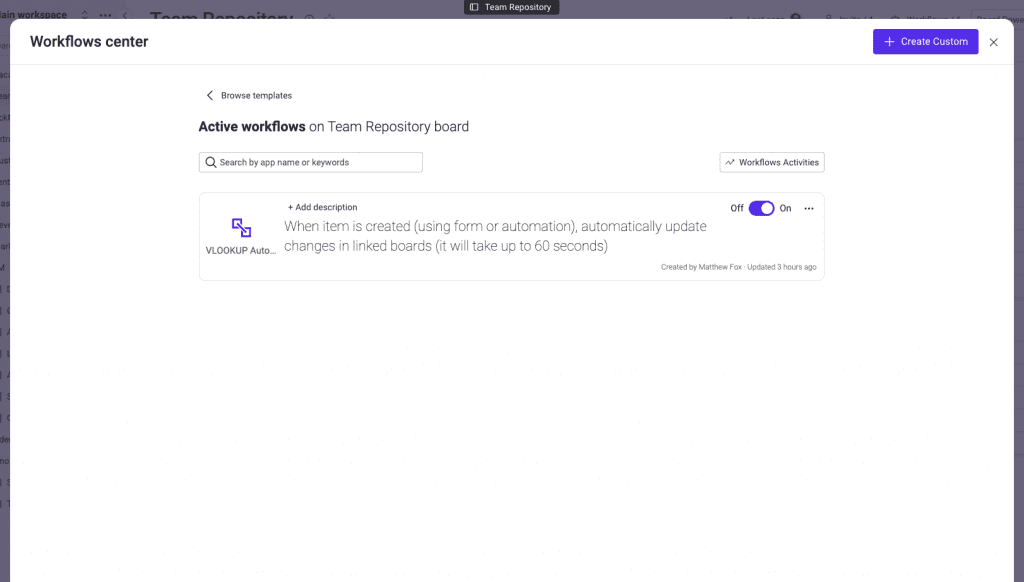The image features a User Interface (UI) screen captured against a white background. At the center, it prominently displays "Workflow Center" within a blue rectangle. Below this, there is a "Plus Create Custom" button and a left arrow labeled "Next," followed by a "Browse Templates" option for selecting predefined workflows. 

In an adjacent section, labeled "Team Repository Board," the title "Active Workflows" is bolded, emphasizing its importance. A search bar is located beneath this section to facilitate the easy locating of specific workflows. Following the search bar, the section "Workflows Activities" is displayed, which includes detailed descriptions for various automated actions. These descriptions include, "Add description when an item is created using form of automation" and "Automatically update changes in linked boards," with the note that each action may take up to 60 seconds to complete.

In the middle of the screen, there is a functional toggle bar currently set to "On," allowing automated processes to be enabled or disabled. To the right of the toggle bar, three horizontally aligned dots indicate additional settings or options. The image also contains some status indicators or debugging information stating "Created Something False, Marathon False."